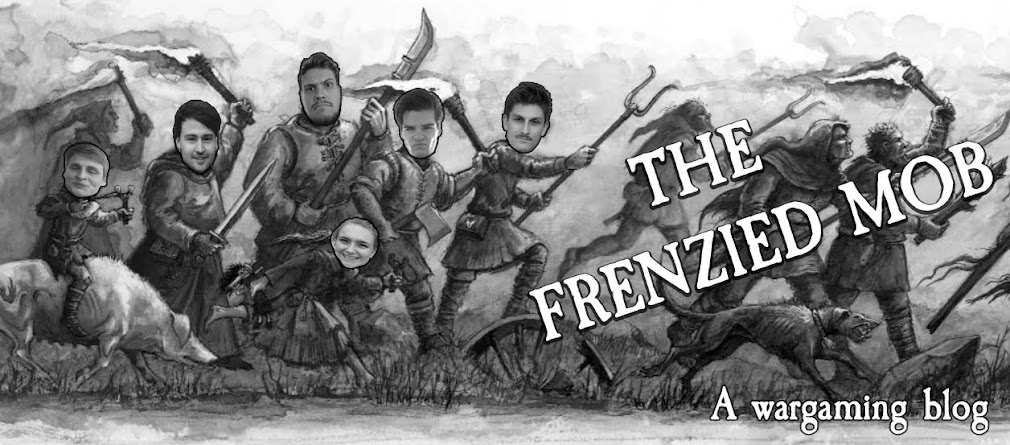The image serves as the front page for a blog titled "The Frenzied Mob," which is a wargaming blog. The banner is a black and white, partially animated composite featuring a humorous medieval scene. It depicts a group of drawn characters arrayed in an assortment of weapons like swords, torches, axes, and skis, marching from left to right. Their faces are replaced with photographs of people, likely representing members of the blogging community. The characters start to the left with more human-like features and gradually transition into caveman-like appearances as they move to the right. Among the group, there is a dog running, seemingly leading the charge, while another dog is shown riding a pig and holding a weapon. The scene is set on a grassy backdrop. The title "The Frenzied Mob" is displayed in bold, white slanted text on the right side of the image, and below it, in smaller white letters, it states "a wargaming blog" against a black background.